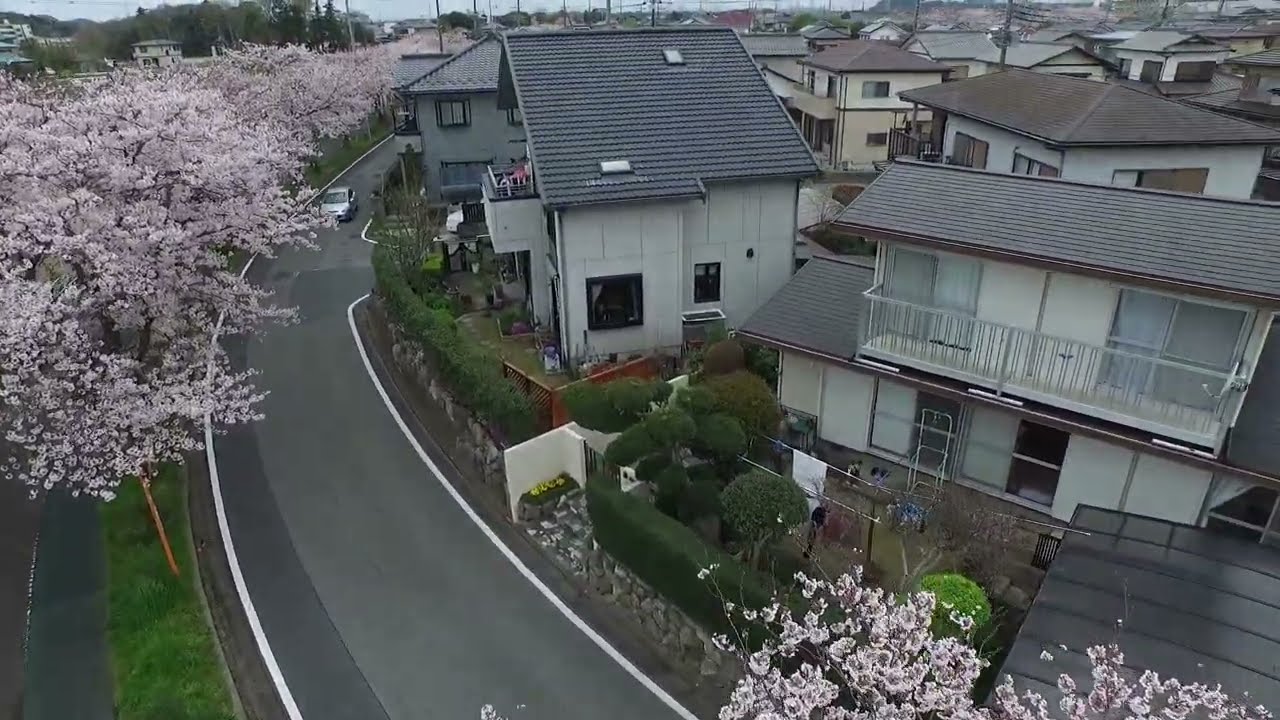This aerial color photograph, taken during the day, depicts a picturesque small residential community from above. The image is in landscape orientation and shows a curved, dark gray roadway starting from the bottom left, winding up to the upper left, and disappearing behind some houses. Alongside the road on the left are cherry blossom trees in full bloom, adding splashes of pink to the scene, and bordered by a grassy area. Toward the right side of the road, there are two-story gray houses with gray roofs and walk-out decks, flanked by green hedges and trees. The houses, predominantly beige and white with variations in roof colors such as brown and gray, dominate the middle to the right side of the image. The roofs of these houses and the tops of various trees, including another flowering tree in the bottom right corner, are clearly visible. The style is realistic and highly detailed, showcasing the serene environment of this suburban setting.